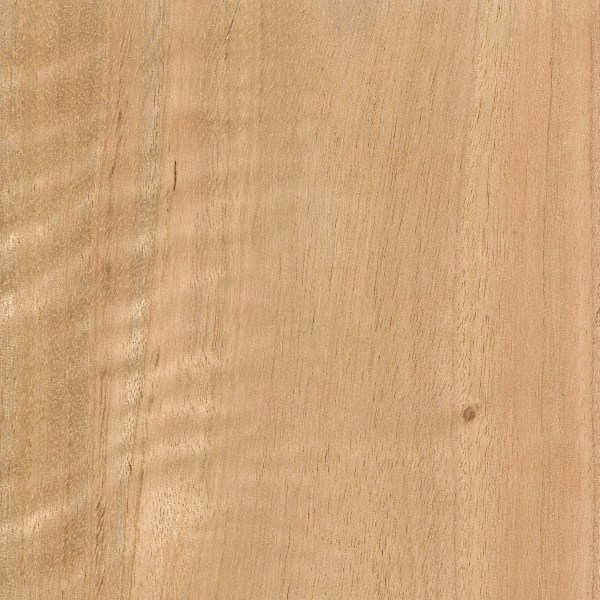This is a detailed, close-up image of a light beige-brown timber panel. The photograph captures the fine lines and grains of the wood, showcasing intricate details and natural imperfections. On the right side of the image, about one-third of the way up, there is a small, dark brown knot beginning to form. The left side features a slightly darker discoloration, almost unnoticeable unless closely inspected. The wood grain exhibits a subtle rippling pattern with occasional darker brown slits. The overall lighting highlights the texture, creating a realistic depiction of the timber's surface.